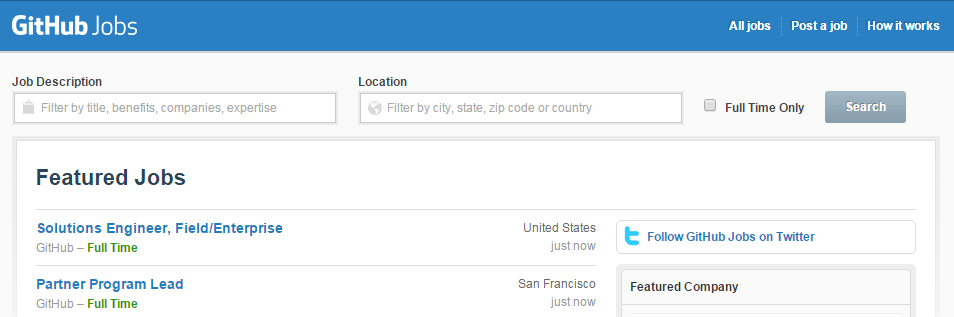This image captures a screenshot taken from the GitHub Jobs web page. The topmost section consists of a long, skinny blue rectangle stretching from the left to the right edge of the screen. The text "GitHub" is prominently displayed in white, with the word "Jobs" following in a thinner font.

Just below this title section, there is a navigation bar with several options: "All Jobs," "Post a Job," and "How It Works." Moving further down, the background becomes a very faint gray, contrasting against the white content boxes laid over it.

In the main content area, there's a job search interface. At the top, filtering options are provided, allowing users to refine their search by Title, Benefits, Companies, Expertise, and Location. Specific location inputs can be filtered by City, State, Zip Code, or Country. Additionally, there is a checkbox labeled "Full Time Only," followed by a gray search button with white lettering.

As the page continues downwards, a section titled "Featured Jobs" is visible. Here, various job listings are displayed. One listing is for a "Solutions Engineer, Field/Enterprise," indicated as a full-time position with the job title in green text. Another listing for a "Partner Program Lead" features the title in blue text, while the "full time" status remains in green text.